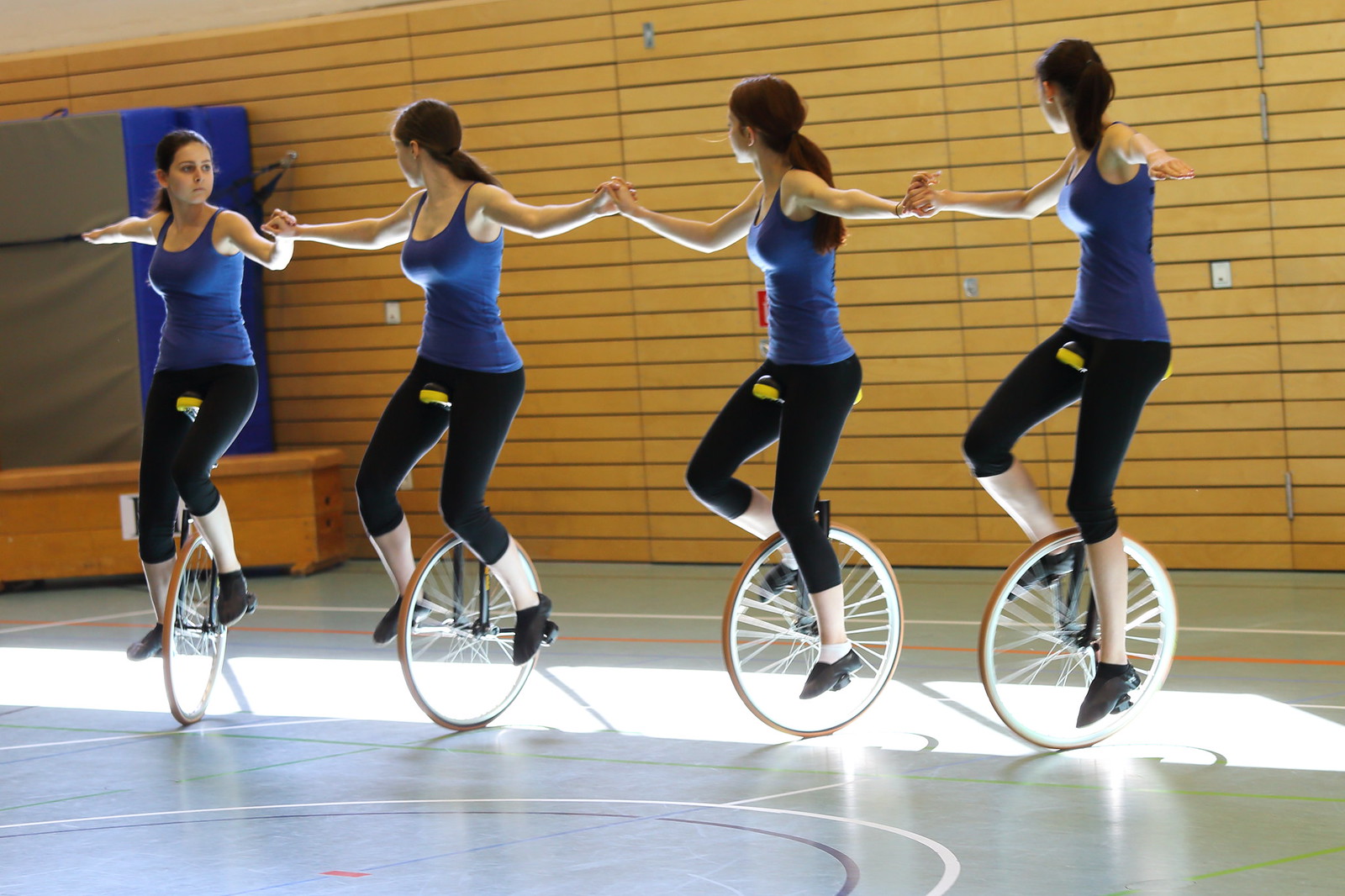The color photograph captures five young women in a gym, each poised on a single-wheeled unicycle. They form a line while holding hands, suggesting a coordinated routine or practice session. Their attire is uniform: black knee-length leggings, blue sleeveless tops, and black shoes. A yellow logo, centrally placed near the crotch area on their leggings, adds a distinct feature to their outfits. All the women have long, straight hair tied into ponytails, mostly low but one higher on the far-right.

The gym setting is evident from the grey floor marked with white and orange lines and curves, hinting at various sports. Behind the women, a wooden-paneled wall, medium brown in color, runs horizontally with an array of power outlets in the middle. On the wall’s left side, a folded large blue and grey mat rests atop a ledge. The gym's environment suggests a multifunctional space, potentially used for different training activities or performances.